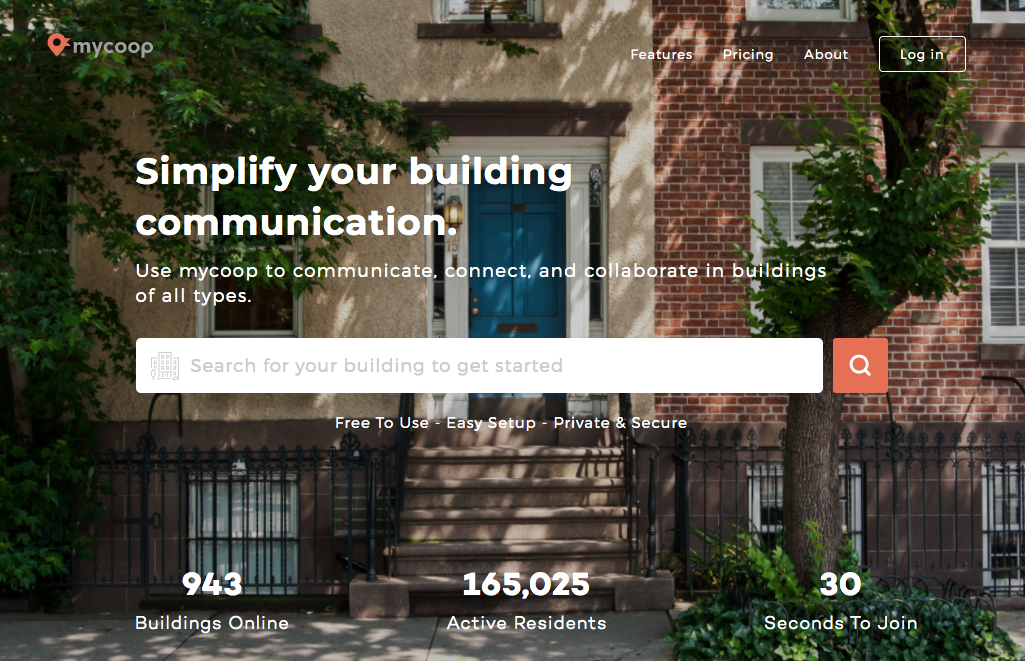The image is a screenshot featuring the interface of MyCoop, a company identified by its name in the top left corner along with a logo resembling a red Google Maps locator icon. Central to the image is a blue door framed by white sides and a lamppost, suggesting the entrance to a house. On the left side of the door stands a tree, while the house's exterior walls have a subtle flesh-toned hue. Leading up to the blue door are six steps.

Prominently displayed in the middle of the image is the text, "Simplify your building communication," in white font. Below this, a detailed tagline reads, "Use MyCoop to communicate, connect, and collaborate in buildings of all types." 

A white rectangular search bar occupies the center, with the placeholder text "Search for your building to get started." To the right of the search bar is an orange, squarish magnifying glass icon meant to initiate the search function. At the bottom of the screenshot, additional text highlights the key benefits: "Free to use, easy setup, and private and secure."